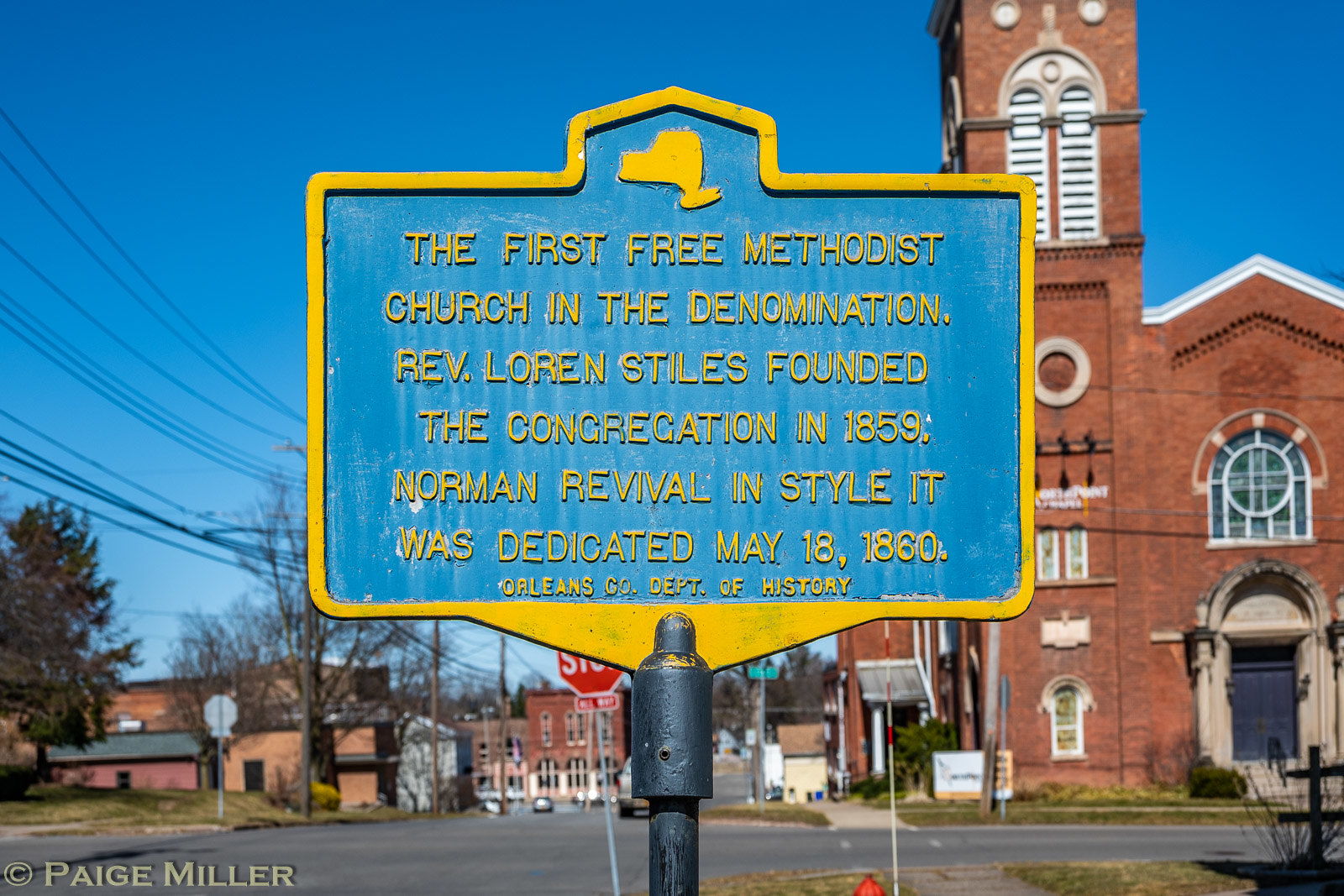The image depicts a vibrant, sunny day with a bright blue sky, showcasing a picturesque scene of a historic red brick church located on the right side. This church features a steeple, though the top is not visible in the image. The church is noted for its Norman Revival architectural style and is identified as the first Free Methodist Church in the denomination, founded by Reverend Loren Stiles in 1859 and dedicated on May 18, 1860. This information is prominently displayed on a rectangular sign mounted on a black-painted metal post in the center of the image. The sign has a blue background with yellow lettering and is bordered in yellow.

The backdrop includes a small community with several brick and possibly vinyl-sided buildings suggesting a mix of office spaces or small businesses. A few cars are visible on the street near a three-way stop, with a partially seen stop sign confirming the location. Telephone lines cross the sky on the left side, and a few trees along with greenish-brown grass add to the scenic setting. The image also mentions the Orleans County Department of History at the bottom of the sign and contains the name Paige Miller in the left-hand corner.